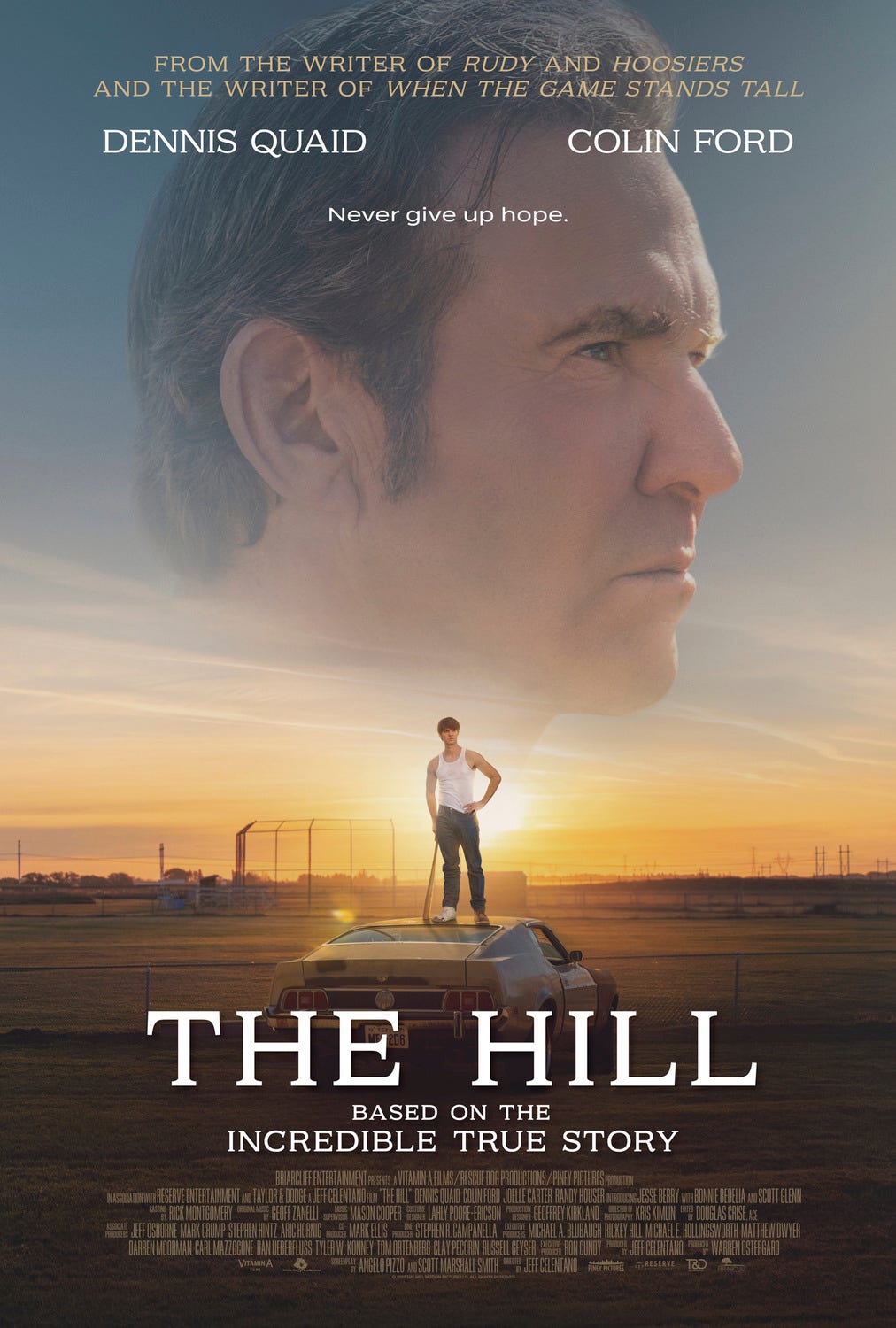This detailed movie poster for "The Hill" features a dynamic and inspirational scene set during a sunset. Dominating the top portion of the poster is a large, contemplative profile of Dennis Quaid's face against an evening sky. Below, a young male, dressed in a white tank top and black pants, stands confidently on top of a classic 70s or 80s muscle car, holding a baseball bat. The surrounding background depicts an empty baseball field. Above Quaid's image, informative text reads, “From the writer of Rudy and Hoosiers and the writer of When the Game Stands Tall.” The actors' names, Dennis Quaid and Colin Ford, are prominently displayed. The tagline, "Never Give Up Hope," is positioned centrally, emphasizing the film's inspirational theme. At the bottom, near the car, the movie title, "The Hill," is stated, along with a note that it is "based on the incredible true story." The poster includes standard casting credits, completing its motivational and evocative presentation.